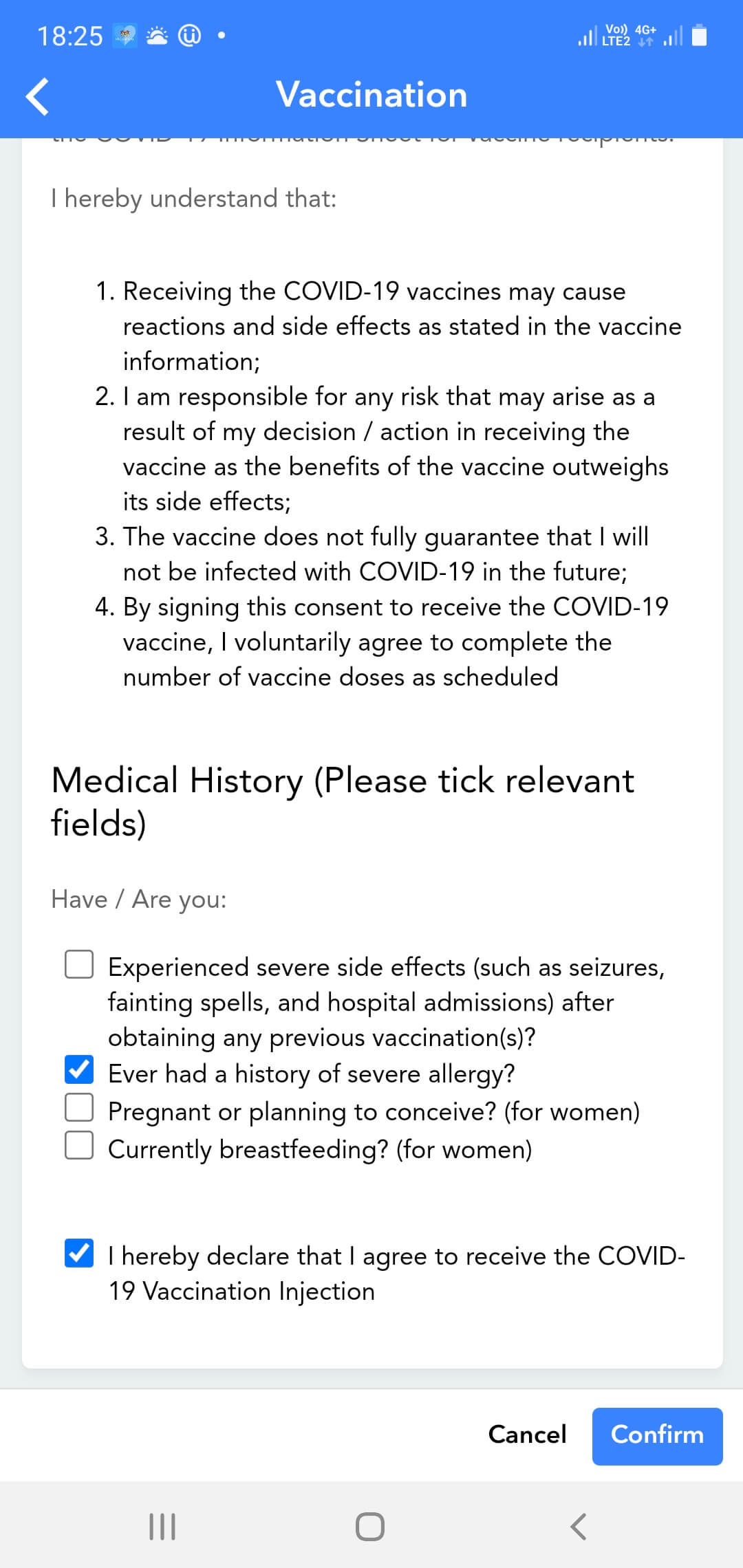**Descriptive Caption**

This is a screenshot from a tablet or smartphone screen. At the top, there is a dark blue, rectangular bezel displaying the time "18:25" in white, without AM or PM indicators. Adjacent to it is a dark blue square containing a blue bubble. Outside of this square, there's a white cloud, a white sun, and a white circle with the letter "U" inside. Additionally, a bold white circle indicates the presence of more notifications.

Directly below, on the left-hand side, a bold white arrow points to the left. Centrally located, the word "Vaccination" is prominently displayed in white text. To the right, signal strength is indicated by a cell phone icon with three white bars and one gray bar. Next to this, the text "VO" appears in white, accompanied by two lines bending to the left, signifying LTE2 and 4G with a plus. Nearby, data transfer is represented by a green down arrow and a gray up arrow, followed by multiple signal lines, including two white and two gray lines. The battery icon, depicted in white, shows it is nearly full.

The main content begins with gray text stating, "I hereby understand that." This is followed by black text detailing the terms and acknowledgments related to receiving the COVID-19 vaccine. These terms include potential side effects, personal responsibility, vaccine efficacy, and consent requirements:

1. "Receiving the COVID-19 vaccines may cause reactions and side effects as stated in the vaccine information."
2. "I am responsible for any risk that may arise as a result of my decision/action to receive the vaccine as the benefits of the vaccine outweigh the side effects."
3. "The vaccine does not fully guarantee that I will not be infected with COVID-19 in the future."
4. "By signing this consent to receive the COVID-19 vaccine, I voluntarily agree to complete the number of vaccine doses as scheduled."

Following this is a bold notice, "Medical History (please tick relevant fields)," along with a list of conditions to check off. Each item is accompanied by white squares with blue checkmarks or unselected white squares with black borders, indicating whether the condition applies:

- "Experienced severe side effects (such as seizures, fainting spells, and hospital admissions) after obtaining any previous vaccinations?" (Unselected)
- "Ever had a history of severe allergy?" (Selected)
- "Pregnant or planning to conceive?" (Unselected, indicated for women)
- "Currently breastfeeding?" (Unselected, indicated for women)

A blue square with a white arrow appears next to the declaration text, "I hereby declare that I agree to receive the COVID-19 vaccination injection."

At the very bottom, beneath a gray border, bold black text offers two options: "Cancel" and a dark blue button with white text stating "Confirm." Below this, there is a mid-gray bezel featuring three black lines, a centered rounded square, and an arrow pointing to the left.